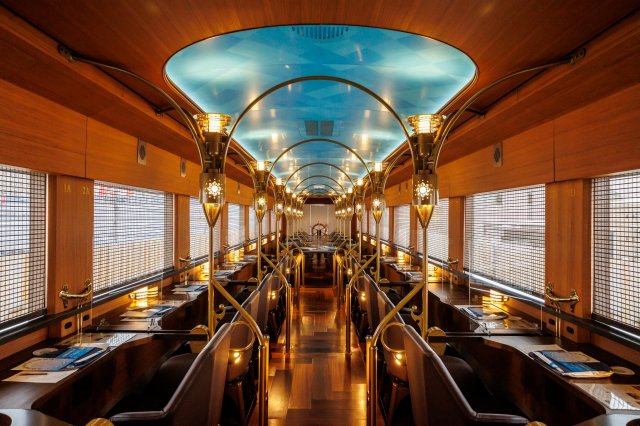The image captures a unique and artistic venue that could be perceived as a luxurious train car lounge, office space, or even a gaming center. The setting is well-lit with a sophisticated ambiance, featuring a high ceiling with a glass skylight running down the middle, flooding the space with natural light. The interior is lined with desks and chairs on both sides, creating individual workspace modules that extend down a central aisle. The design includes interesting and somewhat steampunk-inspired hanging lights, with wooden walls and ceiling, and a light blue section down the middle of the ceiling, possibly with vents. Each workspace is adjacent to a window, enhancing the open and airy feel of the venue. The thoughtful lighting also illuminates the floor, adding to the overall inviting and intelligent atmosphere of the space.